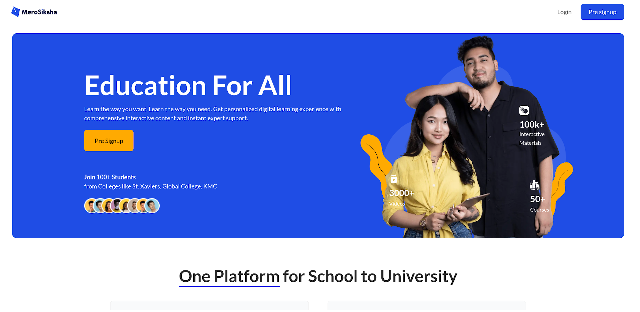This is a screenshot of a university website, featuring a blurred logo at the top left that appears to say "MARC SKHN". On the right side of the header, there are two options; the first likely says "Login" while the second, which is highlighted with a blue background, is unreadable.

Dominating the screen is a large blue rectangular section. On the left side of this section, text reads "Education for all" in white, with further text underneath that is too blurry to decipher. Below this section is a dark yellow bar with additional unreadable text.

Within the blue section, there are several circles with images of people. On the right half, there's a photograph of a man who appears to be of Mexican descent, with light tan skin, short modern haircut, black hair, a thin black mustache, and a small black beard. He is smiling warmly and looks to be around 25-30 years old. He is dressed in a black button-down dress shirt. His arm rests affectionately on the head of a young woman standing in front of him, possibly his daughter. She has long brown hair, a smile that suggests a blend of Asian and Mexican heritage, and is wearing a yellow shirt tied at the front, along with blue jeans. She holds a piece of paper or folder and is wearing a watch on her wrist.

Overlapping the image on his shirt, text reads "100k+" next to something unreadable, and "50+" near his wrist. On the young woman’s right arm (viewer's left), it says "3,000+". Below this blue area is a tagline that reads, "One platform for school to university."